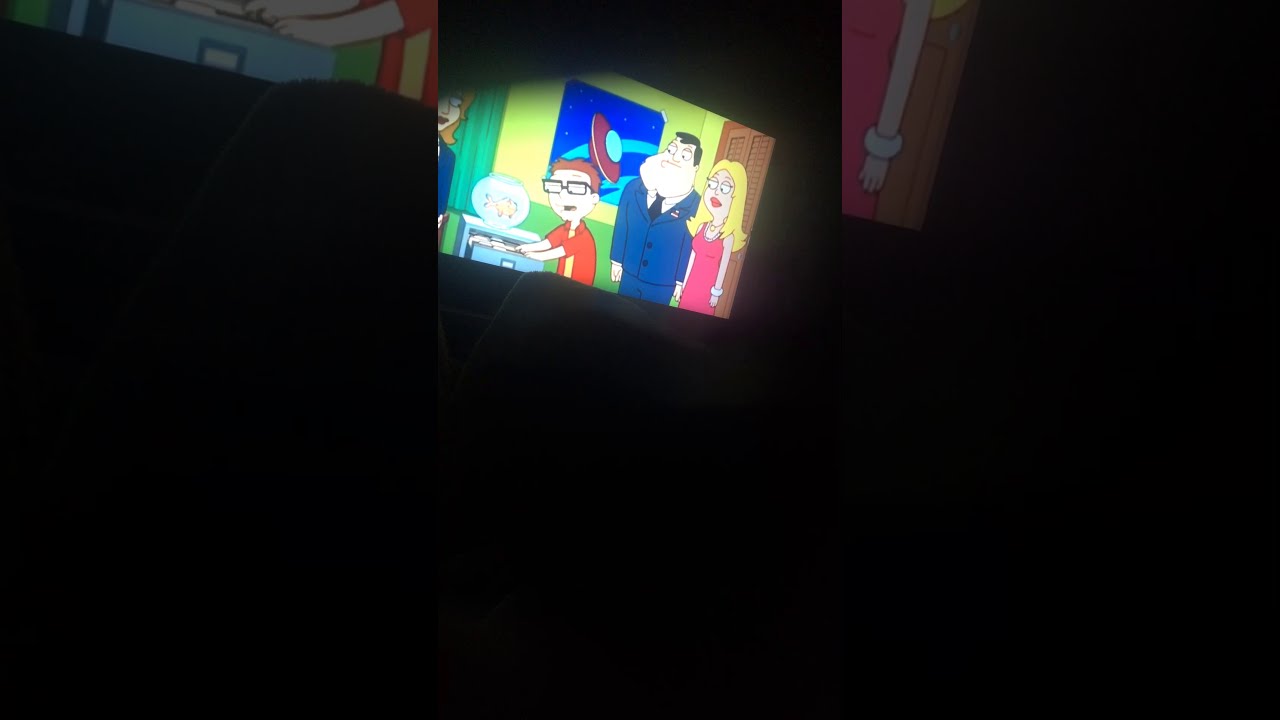In this dark image of a room, the focal point is a TV screen in the upper center, displaying a scene from the animated show American Dad. The TV, which is a modern flat screen, shows a young boy sitting at a desk with a goldfish bowl on it. The boy appears to be interacting with a file cabinet. Standing behind him, the characters of American Dad—Stan Smith in a blue suit and his wife, Francine, in a pink shirt with blonde hair—are looking over his shoulder. The room's background, a yellow-green wall, features a poster that seems to depict a flying saucer. On either side of the main image, towards the margins, are dimly lit red and right-triangle-shaped polygons that blend into the dark surroundings, giving the impression of a less focused background. The image as a whole is characterized by its darkness, making it clear that the scene is likely captured at night or in a poorly lit room.